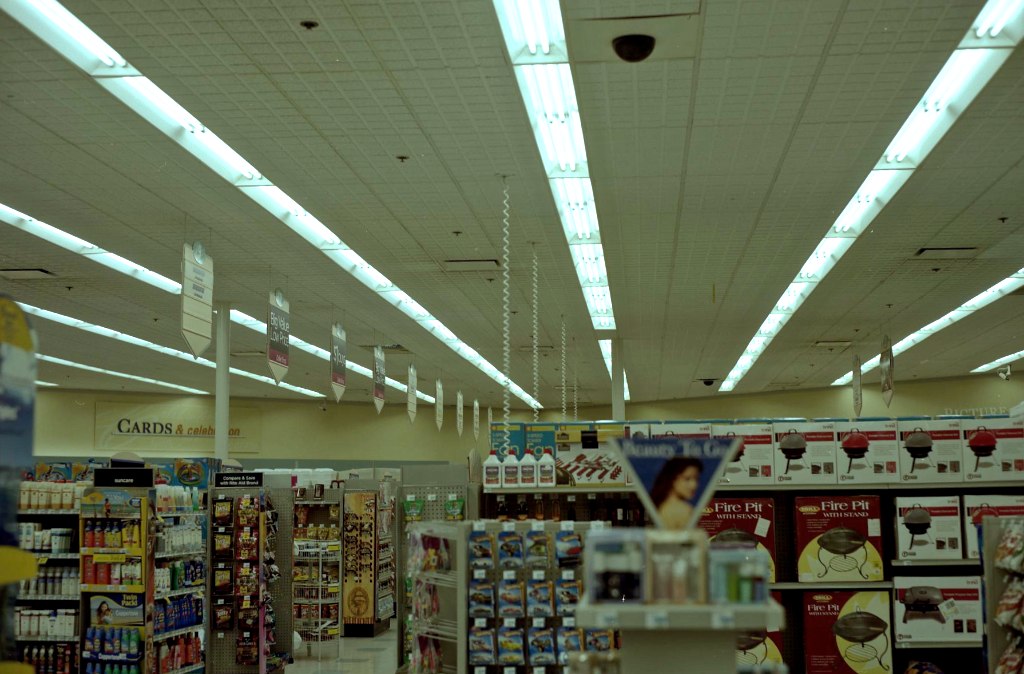The image depicts the interior of a brightly lit supermarket, characterized by rows of shelves stocked with diverse products. Fluorescent track lighting spans across the ceiling, with a pattern of nine layers of lights illuminating the space. Complementing this, the ceiling features an off-white grid design and visible sprinkler systems. Security cameras are also present, with one prominent black-coned camera hanging towards the front of the image and another situated towards the back.

In the foreground on the right, there are tabletop grills and fire pits. The left side showcases rows of sunscreens, with potential snack items positioned further back, although they are too distant to be distinctly identified. A notable sign reading "cards and celebration" is partially obstructed by a support pole on the back left wall, set against pale yellow-colored walls. Additionally, various banners hang above the aisles, contributing to the organized layout of the store. The view appears to be taken from a height of approximately nine feet, offering a clear vantage over the middle section of the shelves.